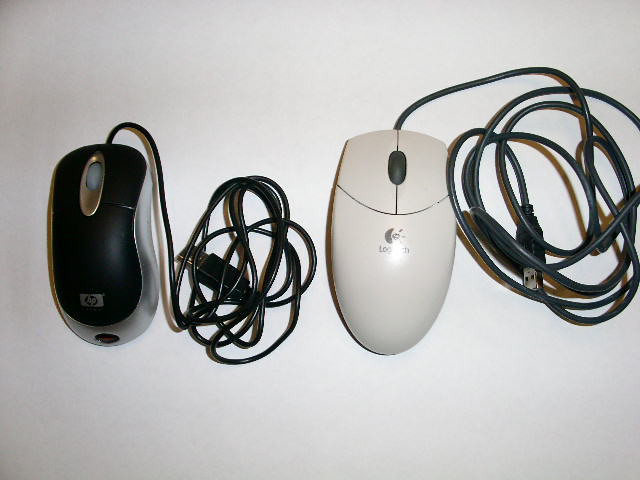A detailed overhead photograph captures two computer mice placed on a white backdrop. The mouse on the left is slightly smaller and features a modern design. It is predominantly black with reflective silver steel ridges. At the top center, it showcases a gold section with a white dot beneath the light gray roller. The bottom of the mouse displays the HP logo in light gray. Its black cord is loosely coiled beside it. 

To the right lies a slightly larger, off-white mouse that has a smoother, rounded shape and appears less ergonomically designed. The middle of this mouse bears the Logitech logo, partially obscured by the lighting. It features a dark gray roller in the center, and its dark gray cord is less tightly wound compared to the other mouse. Both mice rest on a plain white surface.